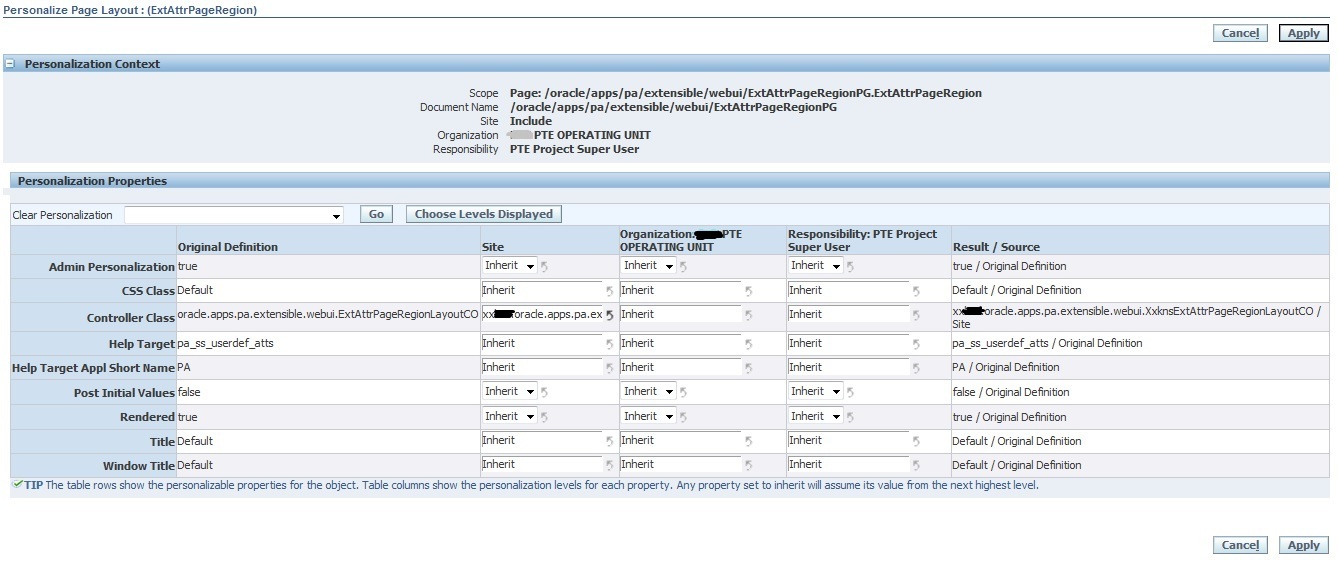This image features a computer screen displaying a personalized page layout interface for a PTE operating unit. The interface includes options for personalization, such as "Personalization Presentation" and "Personalization Properties." It has settings that can be customized to suit the user's preferences and needs. The layout shows two main buttons: "Cancel" and "Apply," allowing users to either discard or save their changes. The screen is predominantly blue and white, with input fields in white and categories highlighted in blue. The interface appears to contain advanced settings and jargon, making it necessary for users to have a strong understanding of computer language and technical knowledge to effectively navigate and utilize the personalization features.